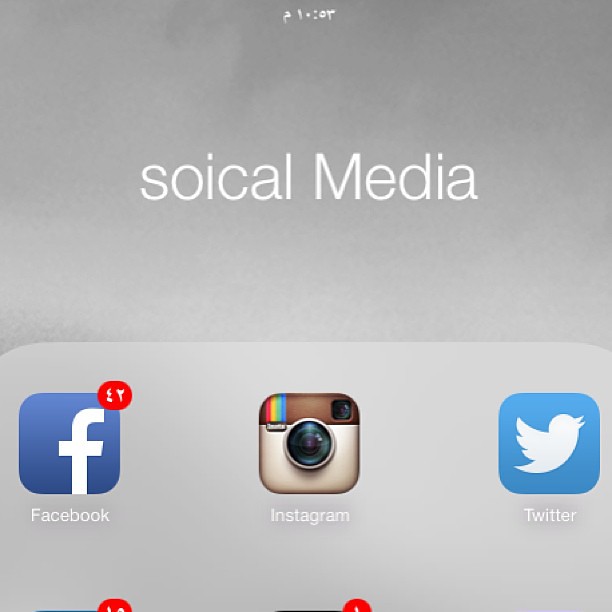The image is a pixelated screen grab featuring a dark gray and light gray background. At the top, in white font, the word "social" is written in lowercase followed by "Media" with an uppercase M. Below this text is a series of social media icons. The first icon is for Facebook, presented in its familiar blue and white colors, with a red notification bubble displaying a white number. The second icon represents Instagram, depicted as a tan camera with a brown strip on top, adorned with red, yellow, blue, and green stripes, and shows a visible camera shutter. Below the Instagram icon, the word "Instagram" is written in white font. The third icon is for Twitter, featuring a light blue background with a blue bird, accompanied by the word "Twitter" in white font at the bottom of the icon. Below these, there appear to be two additional icons, slightly obscured and cropped off, each featuring a red and white notification bubble. Despite a slight pixelation, the overall image remains relatively clear, presenting a recognizable assortment of social media notifications.